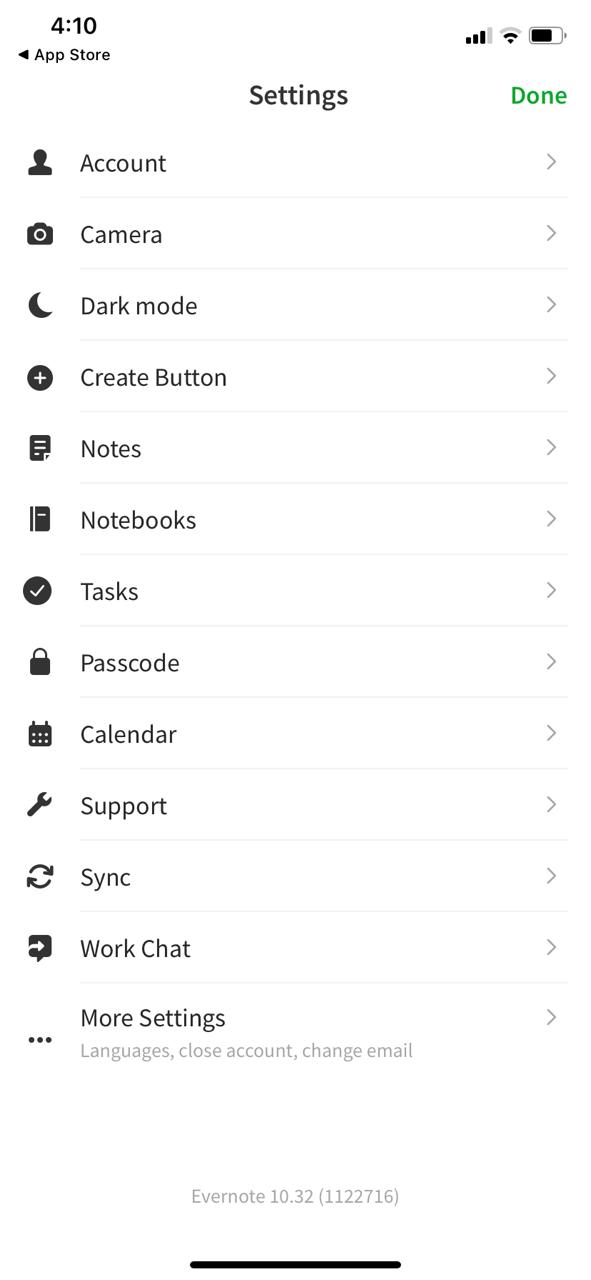This is a detailed descriptive caption for the provided image:

---

The image is a screenshot of what appears to be the settings page of a smartphone, likely an iPhone, given the interface design elements. The top of the screen indicates it's 4:10, with the battery level at approximately 75%. There are two bars showing the Wi-Fi signal strength, and three bars for LTE connectivity. In the top right corner, there is a green "Done" button.

At the center top, the heading "Settings" is prominently displayed. Below this, the screen lists several menu options, each accompanied by a distinct icon and arranged in individual rows with small, gray right-facing carets (>) indicating that they can be tapped for further options. The menu options are as follows:

1. **Account** - Represented by a silhouette of a person.
2. **Camera** - Indicated by a camera icon.
3. **Dark Mode** - Depicted with a half-moon icon.
4. **Create Button** - Shown as a black circle with a white plus sign (+).
5. **Notes** - No specific icon described.
6. **Notebooks** - No specific icon described.
7. **Tasks** - Shown as a black circle with a white checkmark.
8. **Passcode Lock** - Not specifically described but presumed to have a lock icon.
9. **Calendar** - Not specifically described.
10. **Support** - No specific icon described.
11. **Sync** - No specific icon described.
12. **Work Chat** - No specific icon described.
13. **More Settings** - Under this, specific options like "Languages," "Close Account," and "Change Email" are mentioned, all displayed in gray text.

Towards the bottom, the screen shows the app version as "Evernote 10.32" with additional details in parentheses "(1122716)". Below this text, a horizontal bar indicates either more content can be scrolled to or serves as a visual boundary marking the bottom of the screen.

Each row's text is predominantly black except for the "More Settings" sub-options, which are in gray, adding to the interface's visual hierarchy. The clean and organized layout incorporates intuitive icons, providing a user-friendly navigation experience.

---